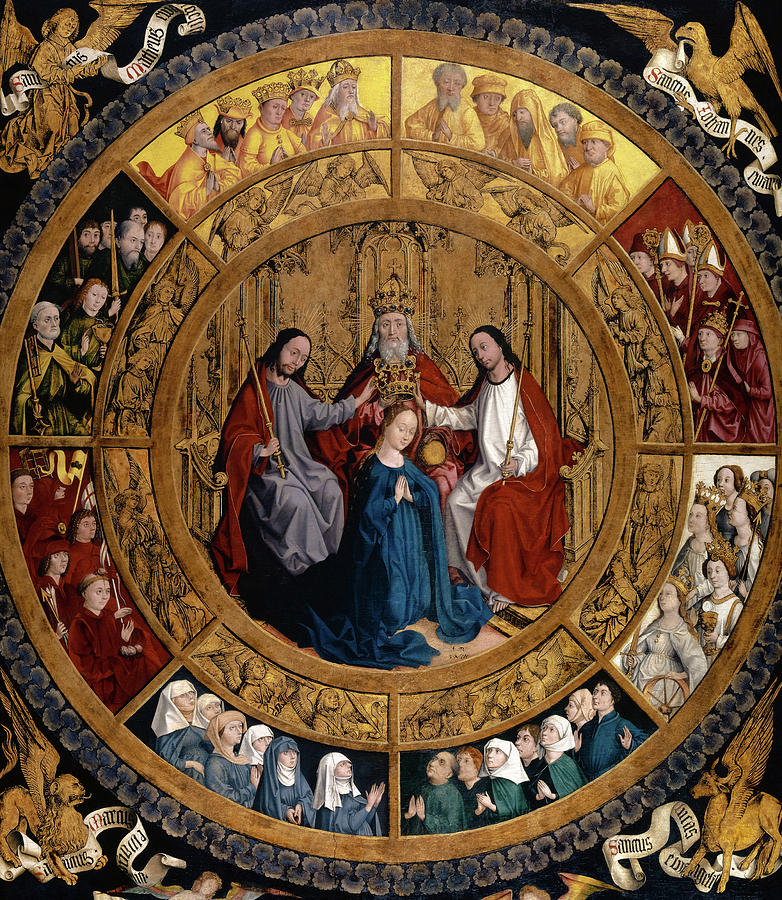This image showcases a detailed and ornate religious scene, likely from an historic art piece reminiscent of a painting found on the ceiling of a cathedral. Central to the composition is a large, elaborate circular frame filled with vibrant and rich colors, predominantly gold, reds, and blues. The scene within this circle appears to depict a coronation ceremony. 

In the focal point of the circle, a woman in a blue robe is kneeling with her hands in a praying position and her head tilted downward. She is being crowned by three men, presumably priests, who are adorned in gold and red robes, each holding staffs with crosses. Behind her, a man in an opulent, gold outfit and crown seems to signify royalty, overseeing the event. Angels with gold wings and various symbolic animals like an eagle flank the scene, adding a divine layer to the imagery.

Surrounding the central vignette is a richly textured background of golden copper hues, filled with intricate scroll-like designs and various groups of figures. On the upper edges, angels and church officials are depicted, while soldiers flank the left and right sides. Below, more common folks and peasants are illustrated, capturing a broad spectrum of societal roles in the religious ceremony. The entire composition is suffused with a majestic and sacred atmosphere, marked by its detailed, historical, and vibrant presentation.